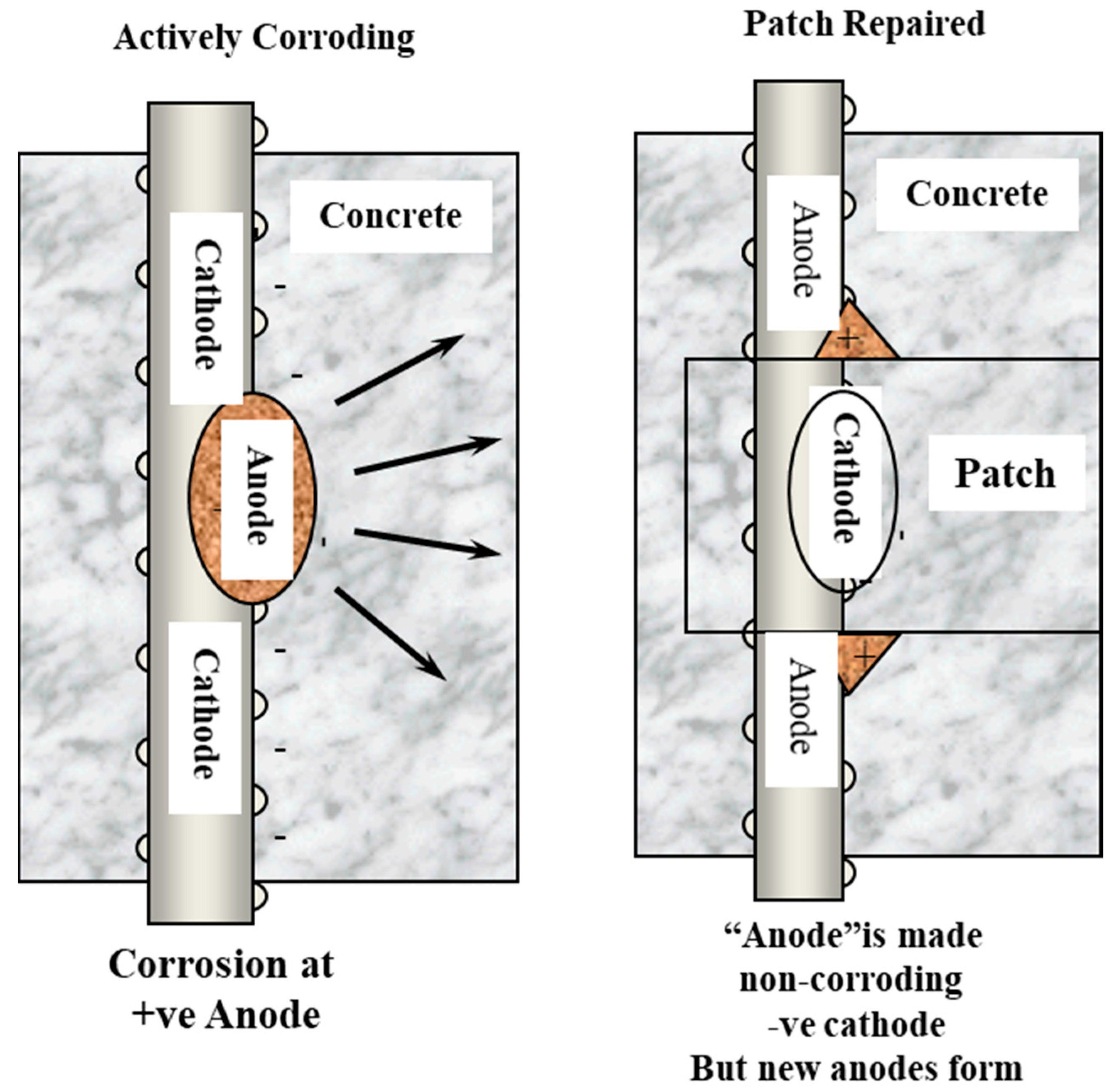This diagram is from an electronics textbook, illustrating the effects of corrosion and repair on concrete structures. The image is divided into two sections. The left side is labeled "Actively Corroding," showing a vertical silver bar embedded in a gray background representing concrete. This bar has a brass-colored anode in the middle, flanked by two cathodes. The anode is marked with positive signs, indicating corrosion, while the cathodes bear negative signs. Below this, there's a label "corrosion at +VE anode."

The right side of the diagram is labeled "Patch Repaired," depicting a similar concrete structure with a central vertical bar. This time, the middle section is replaced by a white circle labeled cathode. It also includes a box labeled "patch" around the cathode area, indicating the repair site. The background is still concrete, and there are new anodes forming, highlighted with positive signs. The text below this image states "Anode is made non-corroding, -VE cathode, but new anodes form." Overall, the diagram details the transition from an actively corroding system to a partially repaired one, emphasizing the interaction between anodes and cathodes in the context of corrosion and repair in concrete structures.